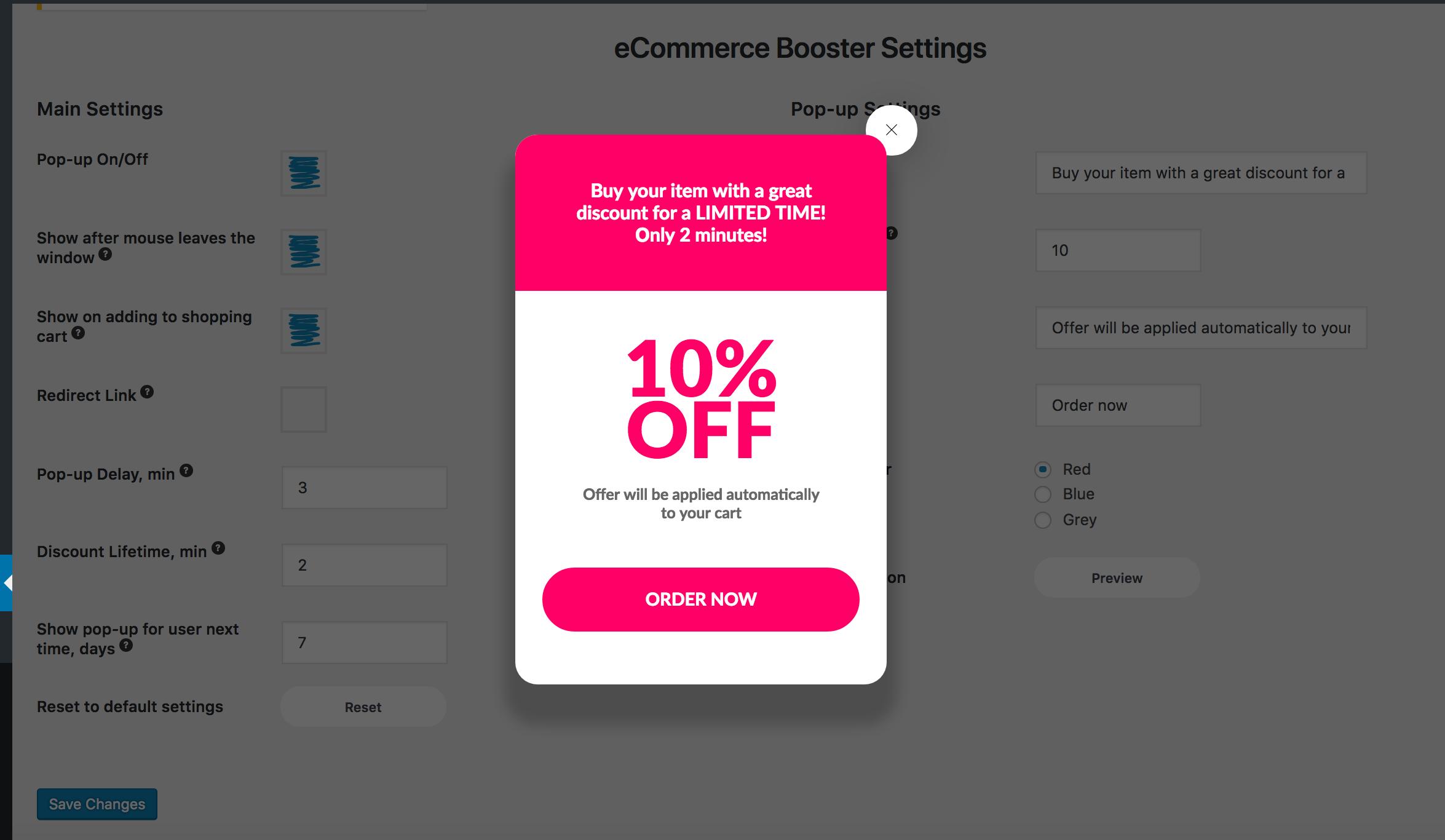The image is a screenshot captured from a web page. Dominating the center of the screen, a pop-up window is prominently displayed. The header of this pop-up announces, "Buy your item with a great discount for a limited time, only 2 minutes." Centrally within the pop-up, bold text advertises, "10% off," and notes that the discount will be applied automatically to the user's cart. At the bottom of the pop-up is a pink "Order Now" button, inviting immediate action.

The background reveals the rest of the webpage, which appears dimmed and darkened, likely due to the focus being on the pop-up. The header of the website reads, "E-commerce Booster Settings." On the left-hand side, there is a vertical menu featuring various settings options—some of which are obscured or scribbled out. On the right-hand side, the user is presented with multiple fields and options, some pre-filled with text like, "Buy your item with a great discount," and "offer will be applied automatically to your purchase." This suggests that the website is likely a configuration page for setting up promotional offers on an e-commerce site.